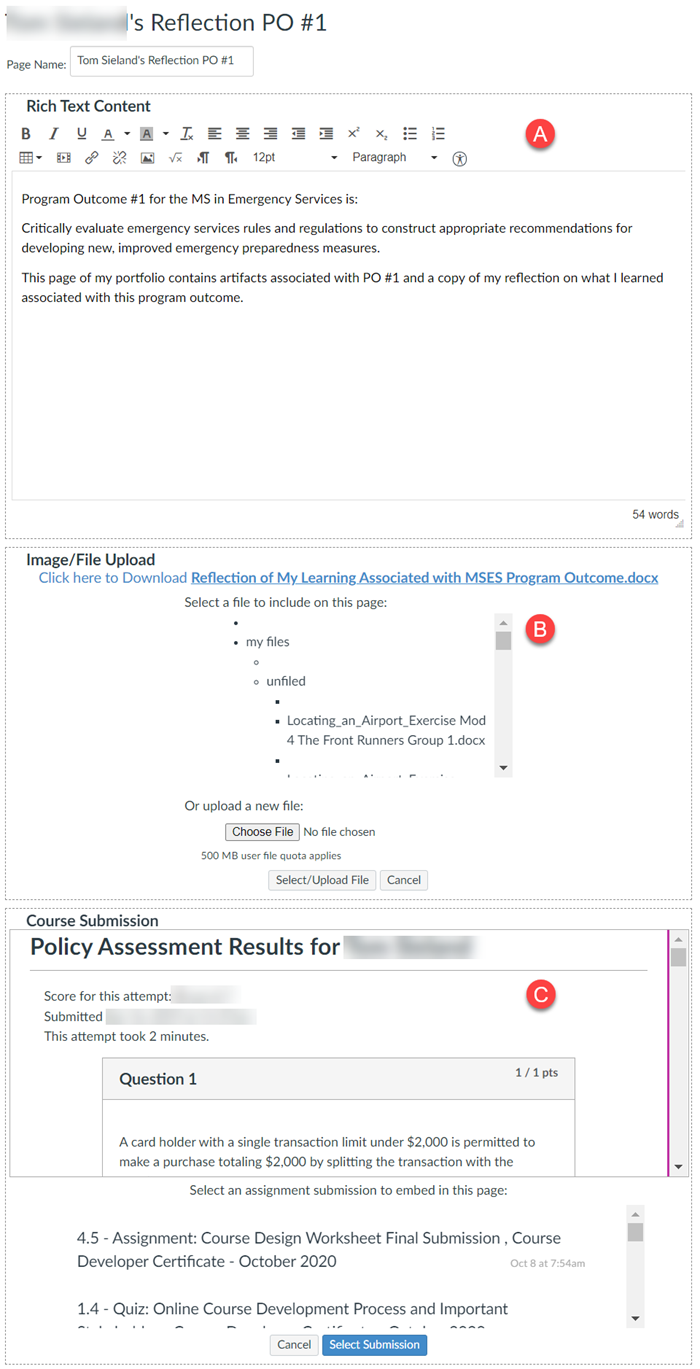Here is a cleaned-up and detailed caption for the described image:

---

The image showcases a web page that appears to be part of an academic portfolio interface. At the very top left corner, there is a text area where a user's name is partially blurred out, only leaving visible the apostrophe 'S' and the text "Reflection PO number 1." Below this, smaller text repeats the page title, stating "Page Name: [User's Name] Reflection PO number 1." This second occurrence of the name is not blurred.

Directly underneath, a section contains multiple thin-lined boxes, mostly rectangular but leaning towards square in shape. These boxes host various UI elements related to text formatting, such as bold (B), italic (I), and underline (U). 

In the first text box at the top of the page, a description reads: "Program outcome number 1 for the MS in Emergency Services is to critically evaluate emergency services rules and regulations to construct appropriate recommendations for developing new, improved emergency preparedness measures. This page of my portfolio contains artifacts associated with PO number 1 and a copy of my reflection on what I learned in the associated program outcome." The word count for this description is noted in the lower right-hand corner as "54 words."

Beneath this, there is another labeled box titled "Image File Upload." It includes a clickable link for downloading a document named "Reflection of My Learning Associated with MSES Program Outcome," highlighted in blue. Below it, there is an option to "Select File to Include in This Page," accompanied by a list of bullet points and a scrolling bar. The bullet points, marked by a circular red "B," list "My Files" (which is empty), "Unfiled" (also empty), and "Locating an Airpoint Exercise Mod for The Frontrunners Group.doc."

Further down, there is a button labeled "Choose File" with the text "No file chosen," alongside options for "Select Upload File" and "Cancel."

The next box is titled "Course Submission." It mentions "Policy Assessment Results" for another blurred name, detailing a "Score Attempt for [Blurred Name]." This attempt clocked in at "two minutes" with "Question 1, 1 out of 1 points."

Inside this box, a cardholder detail reads, "A cardholder with a single transaction limit under $2,000 is permitted to make a purchase totaling $2,000 by splitting the transaction with the..." but the text is cut off here.

Below this is another box that provides an option to "Select an Assignment Submission to Embed into This Page." This section lists:
- "4.5 Assignment Course Design Worksheet Final Submission, Course Developer Certificate, October 2020"
- "1.4 Quiz Online Course Development Process and Important..." (text cut off)

At the bottom of the scroll bar are two buttons: one grey "Cancel" button on the left and a blue "Select Submission" button on the right.

---

This detailed caption outlines the structure, content, and specific UI elements visible on the web page in the image.